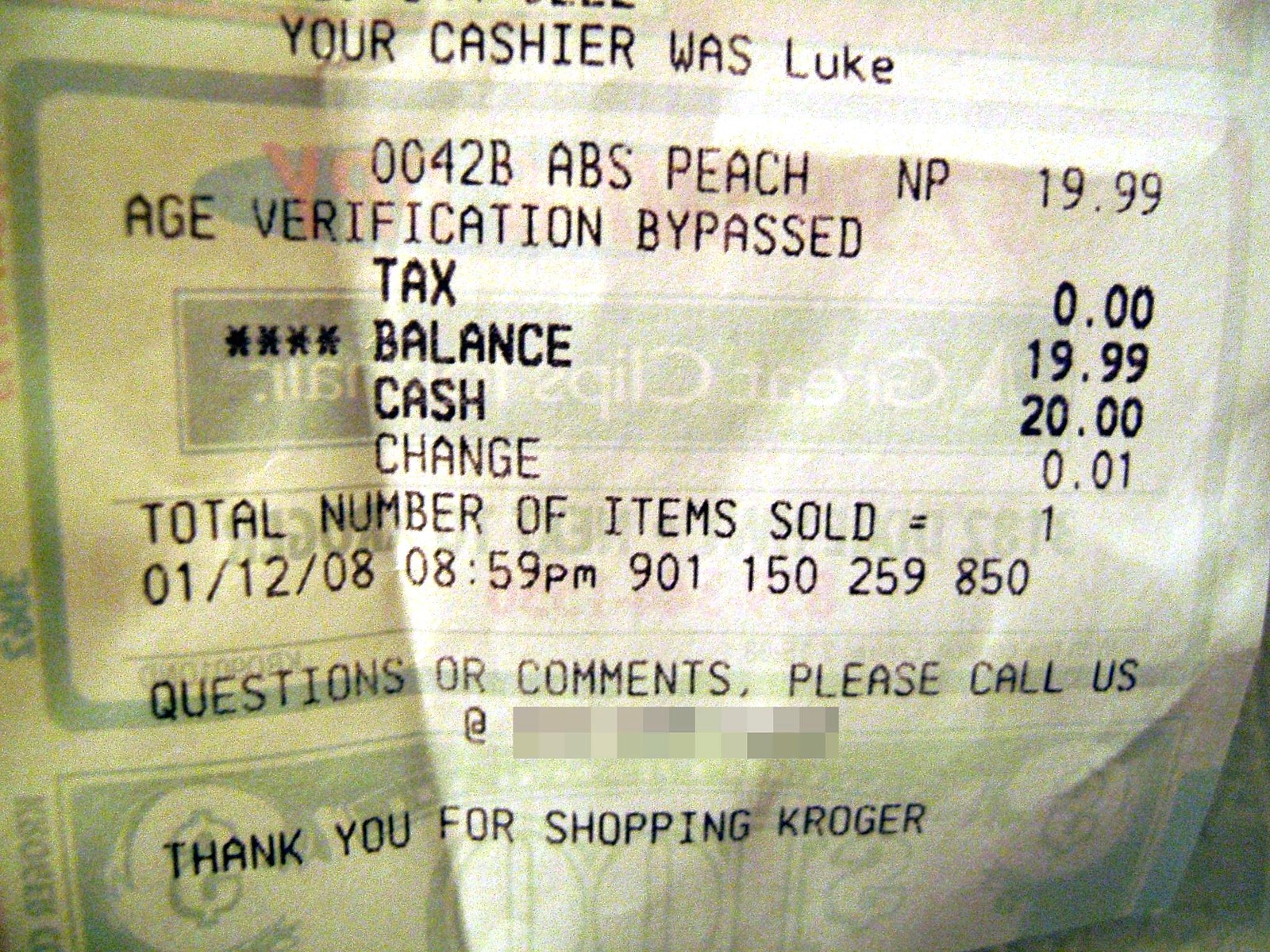Detailed Caption: 

This image depicts a receipt, prominently featuring black text. The top of the receipt indicates that the cashier's name was Luke. The transaction includes the item code "0042B ABS Peach NP 1999," suggesting a purchase of an item labeled as 'ABS Peach NP' with a price of $19.99. An "age verification bypassed" note is visible, implying the item may have age restrictions. No tax was applied, making the total balance $19.99. A cash payment of $20.00 was made, resulting in a change of $0.01. The receipt further indicates that only one item was sold during this transaction. The date at the bottom reads 01/12/08, and the time of the transaction was 08:59 PM.

A string of numbers appears next, reading 901150259850, likely an internal reference or transaction code. The receipt includes a partially blurred-out customer service phone number following an invitation to call with questions or comments. The concluding message thanks the customer for shopping at Kroger.

Behind the primary text, several watermark elements are faintly visible, including text stating "Great Clips" and a pattern resembling a dollar sign and "$100." Additionally, the bottom right corner of the image shows a hint of a blue object, possibly a blanket or similar item.